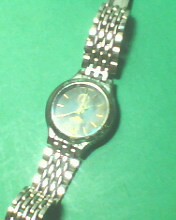This photograph showcases an elegant silver wristwatch with a chain-link band. The watch face appears to be green, although this might be due to the lighting. The hour markers are depicted by short, vertical yellow lines, while the watch hands also exhibit a yellowish hue. The time displayed is approximately 1:40. The watch face is framed by a sleek silver or metallic bezel. The backdrop of the image is a vivid bright green, with noticeable light reflections on the left side of the watch, adding a dynamic touch to the composition.